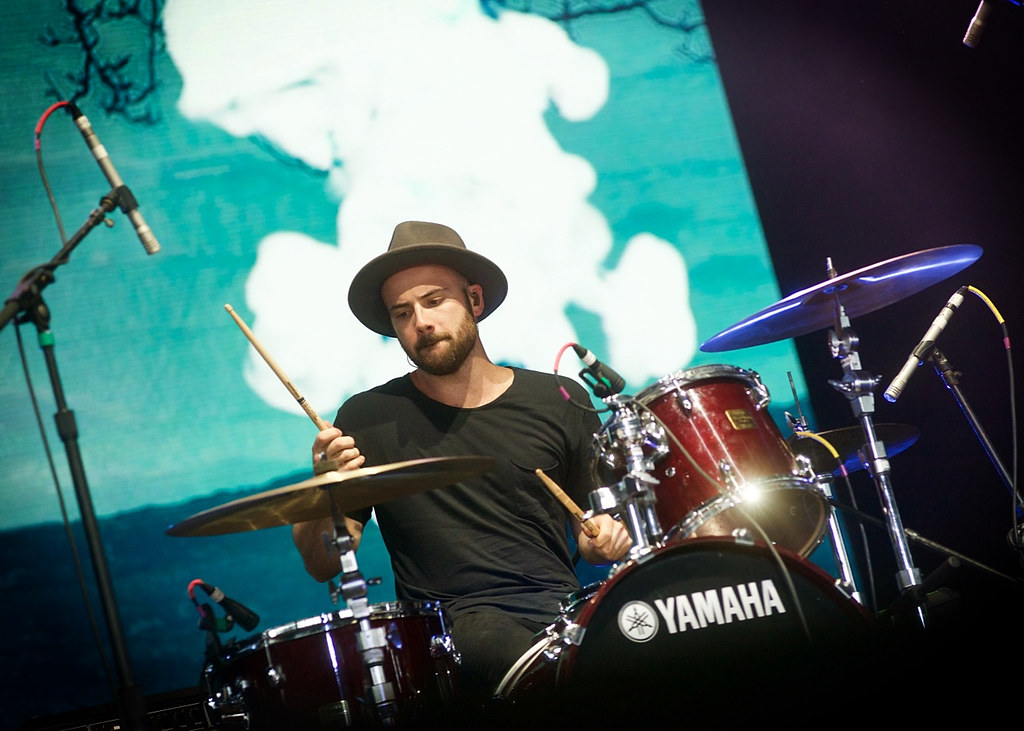The photograph captures a drummer mid-performance, poised to strike with both light wood-colored drumsticks raised. The musician is depicted from the waist up, clad in black pants and a short-sleeve black t-shirt, with a brown fedora perched on his head. His serious expression focuses intently on his red drum set, prominently featuring the Yamaha logo in large white letters on the bass drum. Surrounding him are an array of cymbals and a microphone stand to the left. The backdrop consists of a blue projection screen showcasing an image of a blue sky with blue ground and white clouds, suggesting a concert or stage setting. The drummer sports a black beard, completing his ensemble with a sense of intensity and dedication to his craft.